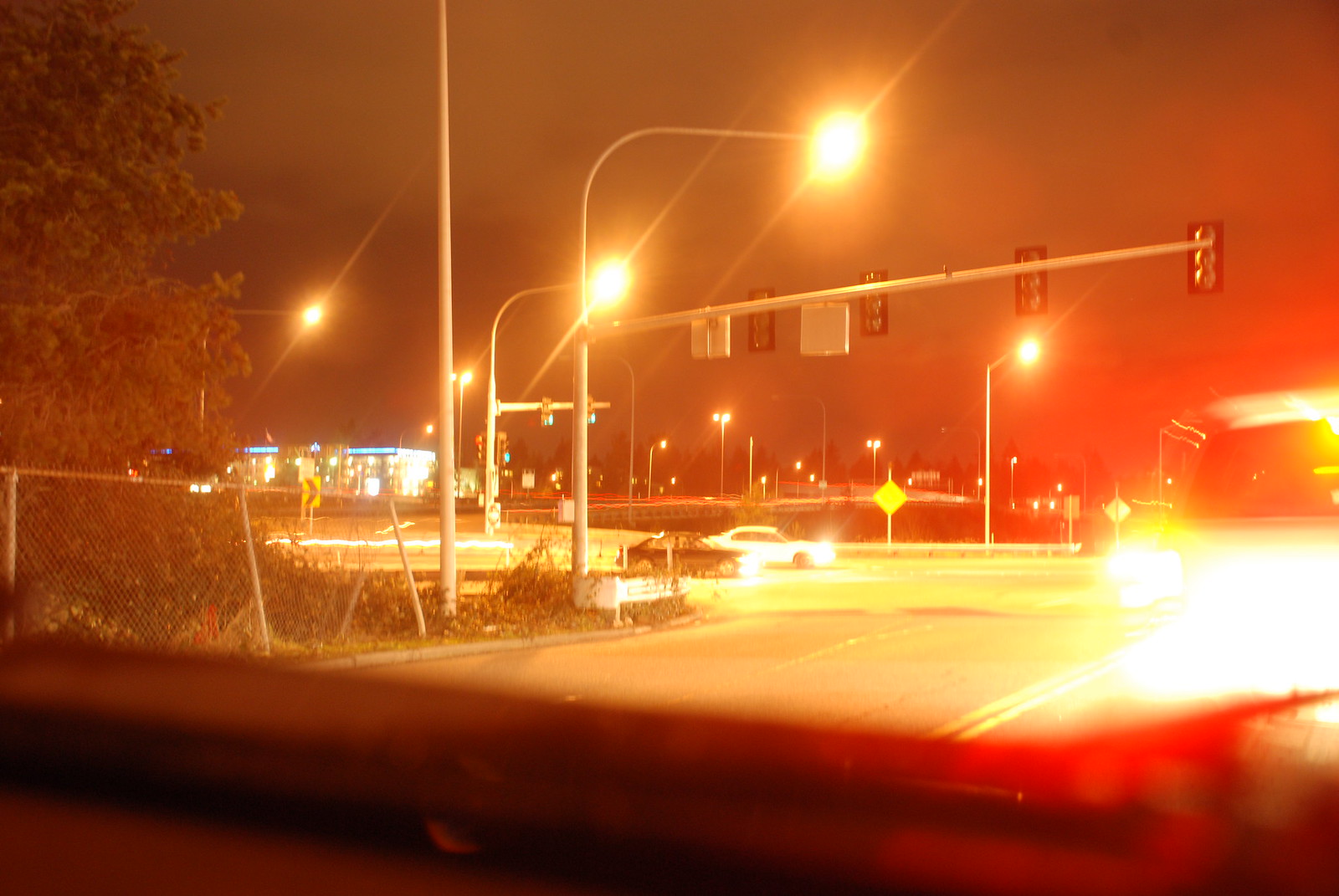A nighttime photograph captures a dynamic street intersection, where the lights create a lined, blurred effect due to the movement and exposure settings. Central to the image are four vertically aligned stoplights, prominently displaying a red signal to the driver from whose perspective the photo is taken. Framed by the car window, the viewpoint includes a partial glimpse of the vehicle's interior. Ahead, another car is seen in motion, its lights and shape also blurred, emphasizing the sense of speed and activity.

To the left of the main intersection, a side road intersects, with two cars making their way through. The background is dotted with several streetlights, their bright yellow illumination diffused into a hazy glow. A business sign with blue lettering sits in the upper left-hand corner, though the details remain indistinct. On the left side, bordering the street, some undeveloped land features patches of shrubbery, providing a stark contrast to the surrounding urban elements. The overall scene captures the nocturnal hustle and bustle of an active city intersection.